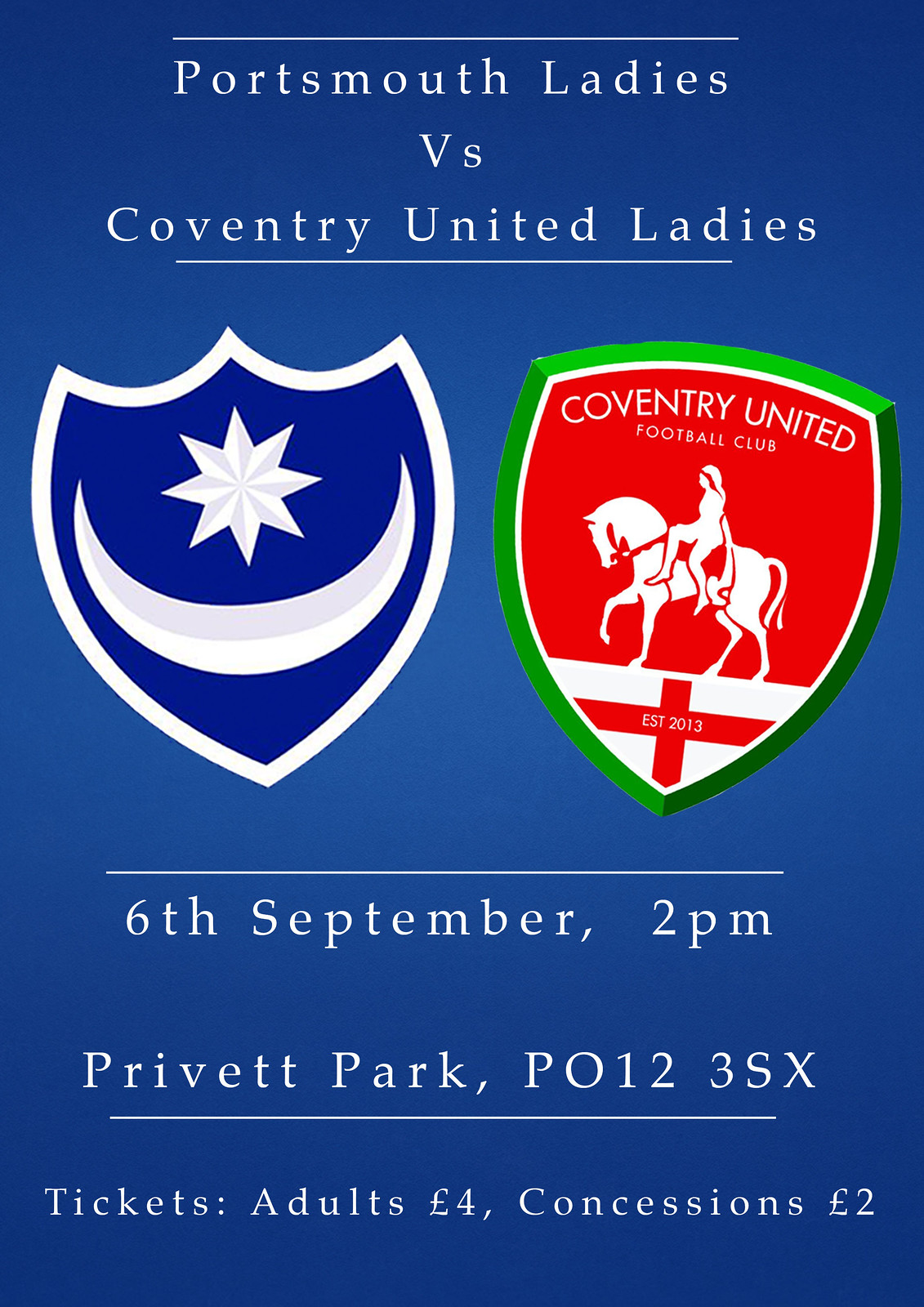This image is an advertisement for a ladies' football match featuring Portsmouth Ladies versus Coventry United Ladies. At the top, the sign has a blue background with white letters. Below the text are two shields: the left shield, representing Portsmouth, is silver and blue with a blue background, featuring a silver crescent moon positioned upwards and a star in the middle. The right shield, representing Coventry United, is red with a green border, and displays "Coventry United Football Club" in white letters, along with an image of a person, likely Lady Godiva, riding a horse. The shield notes the club's establishment in 2013. At the bottom, in white letters, it indicates the match will take place on 6th September at 2 p.m. at Privet Park, P.O. 12 3 S.X. Tickets are priced at 4 Euros for adults and 2 Euros for concessions. The overall design appears to be computer-generated and quite recent.